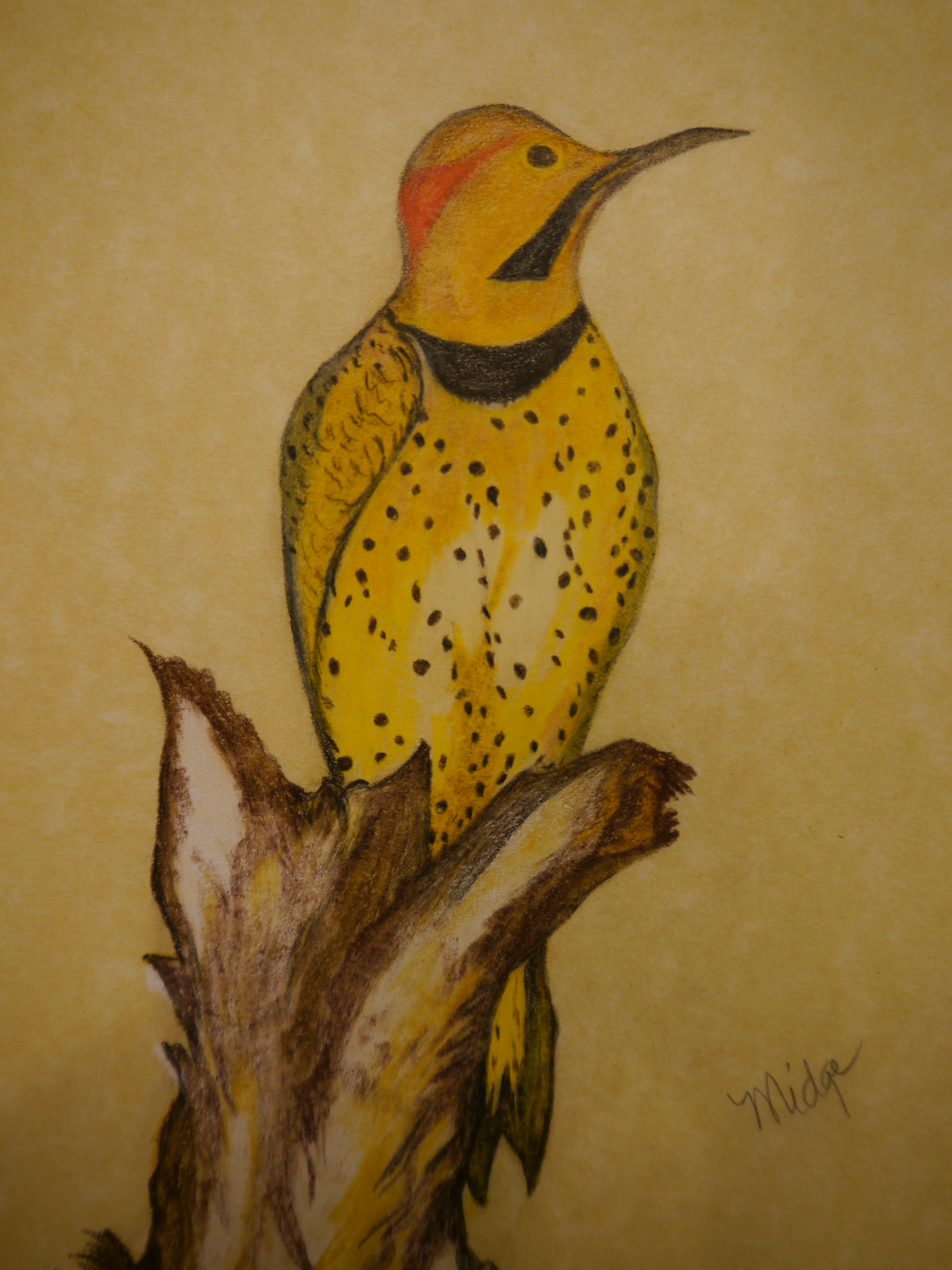This detailed photograph captures a hand-drawn illustration that occupies the entire frame, leaving no visible edges of the paper it was created on. The paper itself appears aged, with a yellowish-white hue that suggests either time-worn patina or intentional coloring to mimic an antique look, occasionally revealing untouched white sections.

The centerpiece of the illustration is a striking depiction of a yellow bird. Its chest and belly are adorned with intricate black specks, reminiscent of a giraffe's pattern. The bird's wings are folded neatly against its body, adding to the sense of calm and containment. Across its neck, there is a distinctive black marking that resembles a bib, adding to the bird's unique markings. The bird's head is predominantly yellow, embellished with a prominent red marking and another black marking that give its face a striking appearance. The bird gazes to the right, its dark gray beak adding depth to the facial details. Its eye is also black, standing out sharply against the yellow.

Perched on a gnarled piece of wood, the bird's setting enhances the scene with an organic, rustic touch. The wood, predominantly brown with patches of the same aged yellow, appears weathered and worn, featuring sharp, twisted textures that add to the illustration's overall character. It seems to reflect some of the bird's yellow hues, creating a harmonious color palette.

In the bottom right corner of the paper, a signature in pencil reads "Midge," elegantly scrawled in cursive, adding a personal touch and crediting the artist behind this captivating piece.